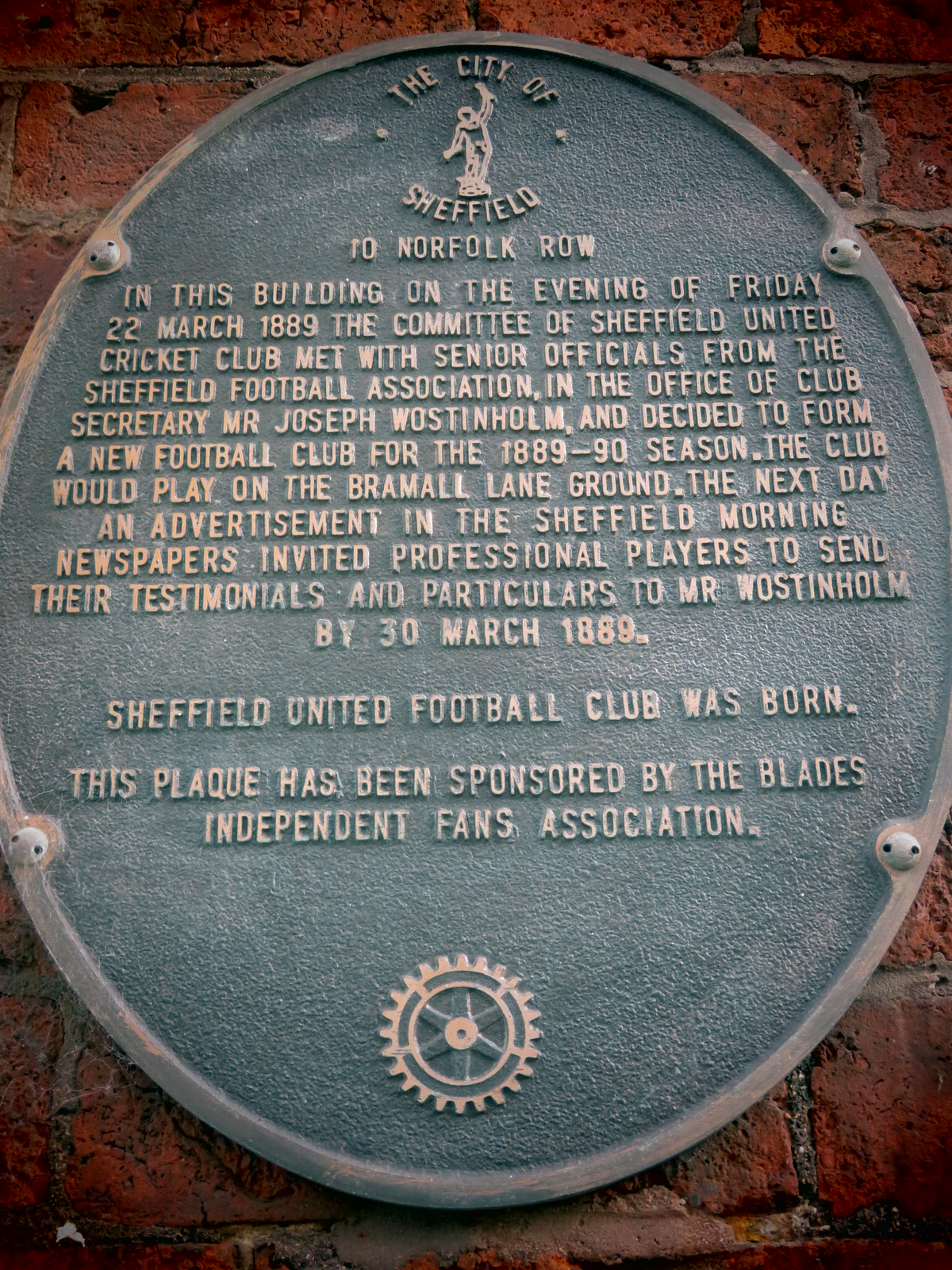The image features an oval, vertically-oriented metal plaque mounted on an aged red brick wall. The plaque, bolted at four corners, has a black textured cast metal background with a border running along its edge. At the top center, it reads "The City of Sheffield, 10 Norfolk Row," with a human figure depicted between the words "City of" and "Sheffield." The inscription details:

"In this building on the evening of Friday, 22 March 1889, the committee of Sheffield United Cricket Club met with senior officials from the Sheffield Football Association in the office of club secretary Mr. Joseph Wostinholm and decided to form a new football club for the 1889-90 season. The club would play on the Bramall Lane ground. The next day, an advertisement in the Sheffield Morning newspapers invited professional players to send their testimonials and particulars to Mr. Wostinholm by 30 March 1889. Sheffield United Football Club was born."

At the bottom of the plaque, a bronze gear wheel is featured. The plaque has been sponsored by the Blades Independent Fans Association, commemorating the historical formation of Sheffield United Football Club.